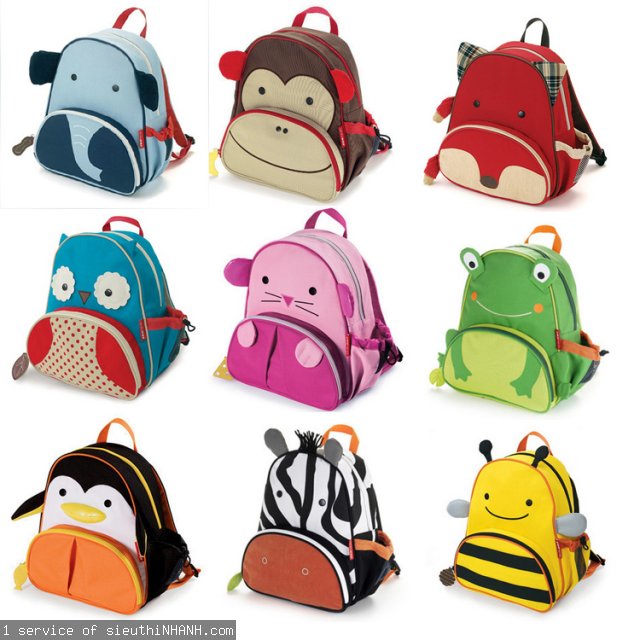This image showcases an array of nine brightly colored and cartoonish children's backpacks, perfect for school. Each backpack is designed to resemble a different animal with playful and cute features, making them ideal for young children. Starting from the top left, the designs include a blue elephant with ears, a brown monkey with ears, a red fox with plaid ears, a blue owl, a pink bunny, a green frog, a black and white penguin with a yellow beak, a striped zebra with a face, and a yellow bumblebee. The backpacks are arranged in three neat rows and share a common style, featuring a smaller front pocket and a larger main compartment, both secured by zippers. They also include a handle and shoulder straps for easy carrying. Additionally, the bottom left corner of the image displays the web address OneServiceOfSeaYouthN9.com, spelled out as S-I-E-U-T-H-I-N-H-A-N-H.com.